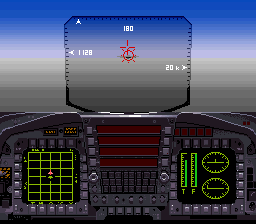This image is a detailed screenshot from a retro video game, depicting the cockpit of a fighter jet. The scene is dominated by a central console area with various displays and controls. At the top, a blue strip symbolizes the sky, indicating that the jet is flying above the clouds. Centered in front of the viewer is a transparent glass rectangle with black tick marks and white arrows along its edges, displaying numbers such as 1128 on the left, 180 at the top, and 20k on the right. In the middle of this rectangle is a red crosshair targeting another plane, represented by a red circle.

To the left of this main display is a green grid-like screen, presumably a radar, showing different aircraft in the area. The radar has green lines on a black background and features buttons surrounding it. On the right side, another screen with a green display shows two green circles with bars in the middle, accompanied by scale-like indicators labeled 'T' and 'F'. Below the central glass rectangle, the dashboard is filled with gray buttons, orange text screens, and various circular knobs. Notably, there are reddish-orange strips and gray buttons at the bottom center. The heads-up display also shows crucial flight information such as heading, speed, altitude, fuel level, and thrust, creating a comprehensive and immersive cockpit environment.